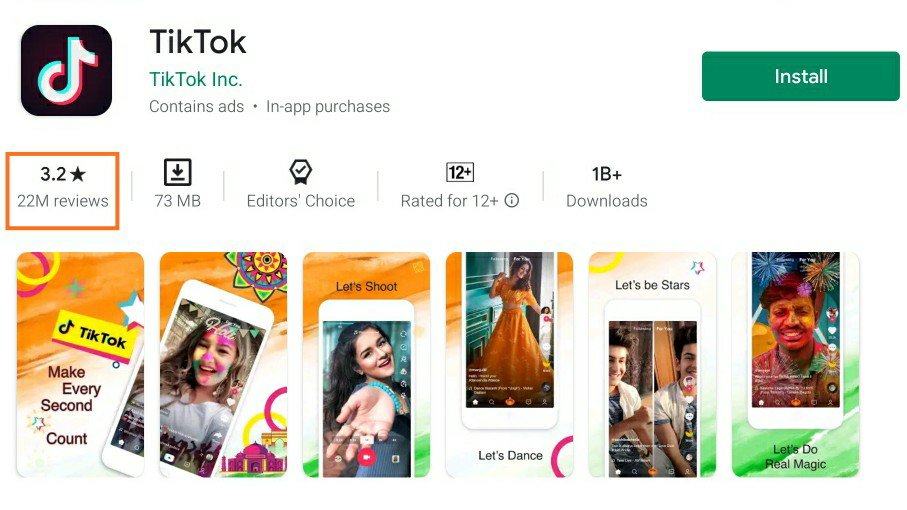This image shows an enlarged view of a page, likely from the Google Play Store, featuring the TikTok app. At the top left corner, the TikTok logo is prominently displayed with "TikTok" in bold black letters and "TikTok Inc." written below in teal green. To the right of the logo, a teal green "Install" button is visible, indicating where users can download the app.

Highlighted within a box on the page is the app's rating of 3.2 stars, based on 22 million reviews. Below this rating section, there are several promotional images, each showcasing the app on different cell phones. In total, there are five cell phone images. Four of these images feature different women, each demonstrating various aspects of the app. The fifth image, with the caption "Let's Be Stars," shows two men standing side by side. 

Additional details on the page include the app's file size, which is 73 megabytes, and a distinguished "Editor's Choice" badge, indicating a high recommendation by the platform.